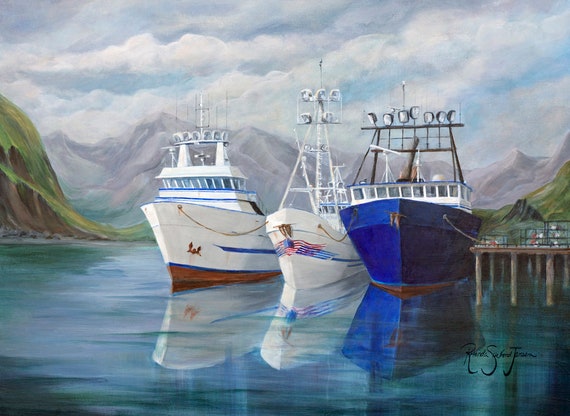The painting beautifully captures a serene lake scene, featuring three medium-sized boats tethered side by side, with the one on the far right also tied to a dock. The boats float placidly on a water surface that showcases a mesmerizing mix of blues, greens, and whites, reflecting the boats’ vibrant colors. In the backdrop, majestic mountains rise under a blanket of daytime clouds, flanked by sweeping hills on either side of the waterfront. 

The boat on the far left is predominantly white with a striking blue stripe above its red bottom. It's equipped with an array of lights atop, suggesting it might be a fishing boat. The middle boat is also primarily white, adorned with a motif of red and blue stripes near the front that bears a resemblance to the American flag. This boat also features lighting equipment. The boat on the right is a rich, metallic ocean blue with a brown trim at the bottom, and it too has lights mounted on top. 

Adding a personal touch to the painting, a signature with initials "R, S, and J" appears faintly on the lower right side, hinting at the artist's identity. Overall, the image radiates a peaceful yet dynamic interplay between the boats, water, and the natural grandeur in the background.